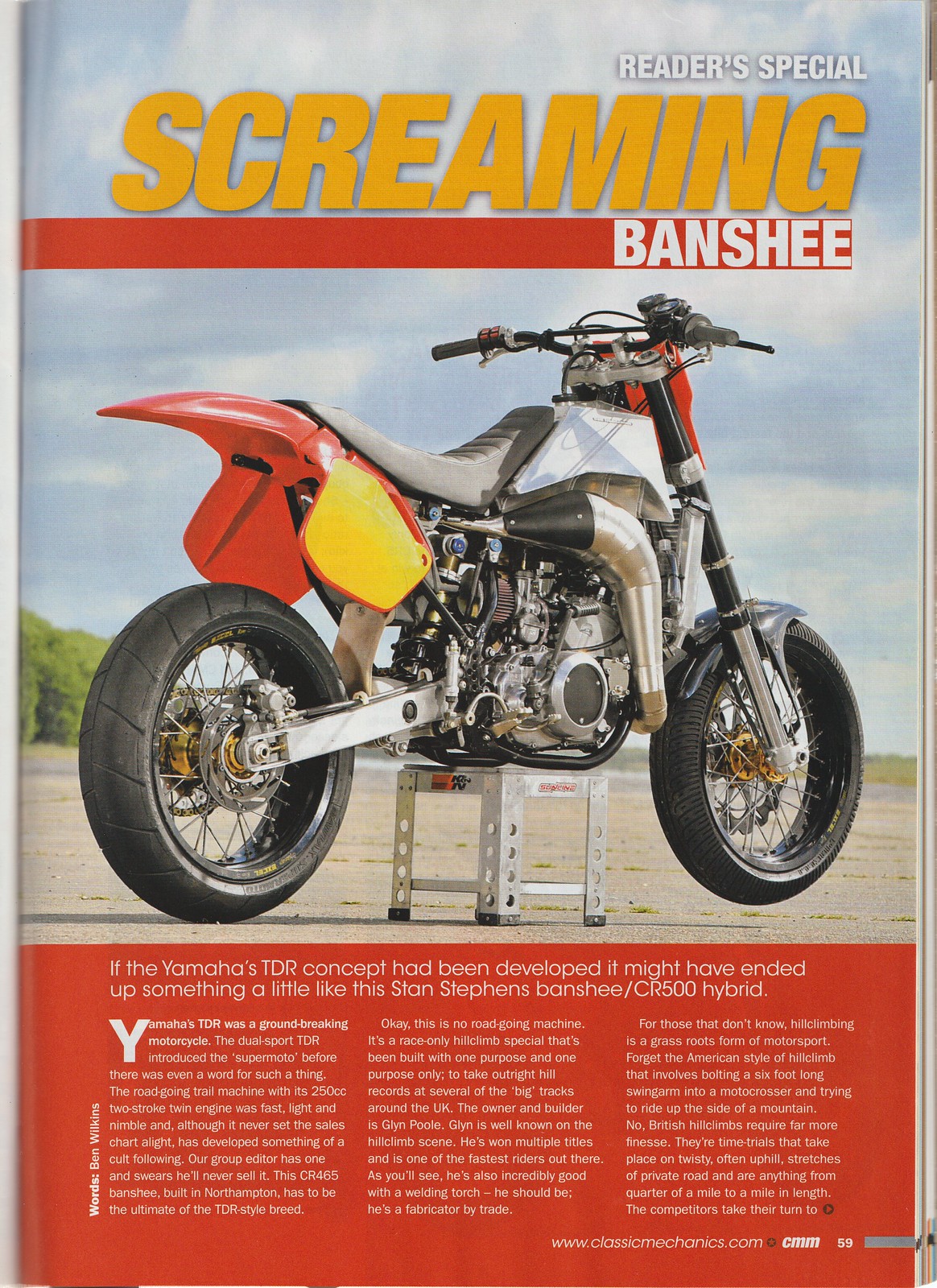The poster features a large side profile shot of a motorcycle prominently displayed in an outdoor, open field setting with trees and a sky filled with clouds, captured during the daytime. The motorcycle, elevated on a metal stand, showcases its striking red fender accented with yellow, a gray seat, black wheels, and a chrome engine. At the top right corner, white text reads "Reader's Special," and beneath it, in yellow font, is the phrase "Screaming" followed by a red bar with "Banshee" in white font. The bottom third of the poster, set against a reddish background, includes the text: "If Yamaha's TDR concept had been developed, it might have ended up as something like the Stan Stevens Banshee/CR500 Hybrid,” with three columns of text below this line. The trees, sky, and predominantly sandy terrain provide a vivid backdrop to the strikingly detailed motorcycle.